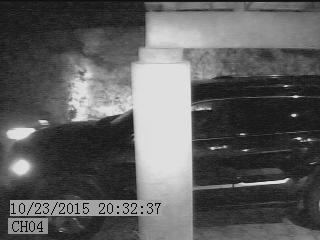The grainy black-and-white security camera image, timestamped 10-23-2015 at 20:32:37, captures a dark-colored SUV with its headlights on, possibly in a parking lot. The vehicle, seen from the driver’s side, is partially obscured by a light gray or white pillar positioned centrally in the frame. Despite the close proximity, the driver is indistinguishable. The background features a nondescript concrete wall and a hedge, indicative of a night setting. Bottom left corner annotations read "channel 4," suggesting the footage is from a local camera feed.